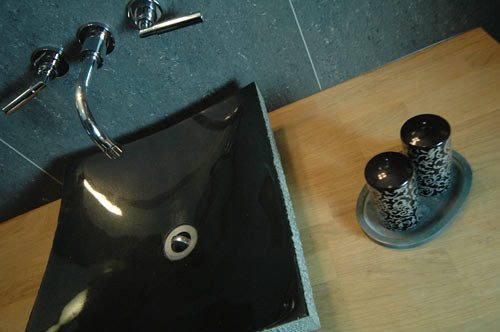This image showcases a modern bathroom sink set against a backdrop of large, gray tile walls. The tiles, which appear to measure approximately 16 to 18 inches square, extend from the upper left to the upper right corner of the image, reflecting some light in the upper left corner. The sink is positioned at an angle, revealing its unique design—a square shape with upturned edges, most pronounced at the corners. In the center of the black sink, there is a silver drain. 

The sink is equipped with chrome fixtures: two separate handles and a centrally placed spout, all gleaming under the light. It rests on a light-colored, butcher block-style countertop, which displays distinct wood grain patterns. 

To the right of the sink, a gray tray holds two canisters with a marble-like pattern in shades of black and white, each topped with a black lid. While the purpose of these canisters is unclear, they contribute to the overall aesthetic of the space. Shadows cast by the canisters stretch towards the sink, hinting at an external light source that enhances the modern and clean design of the bathroom.